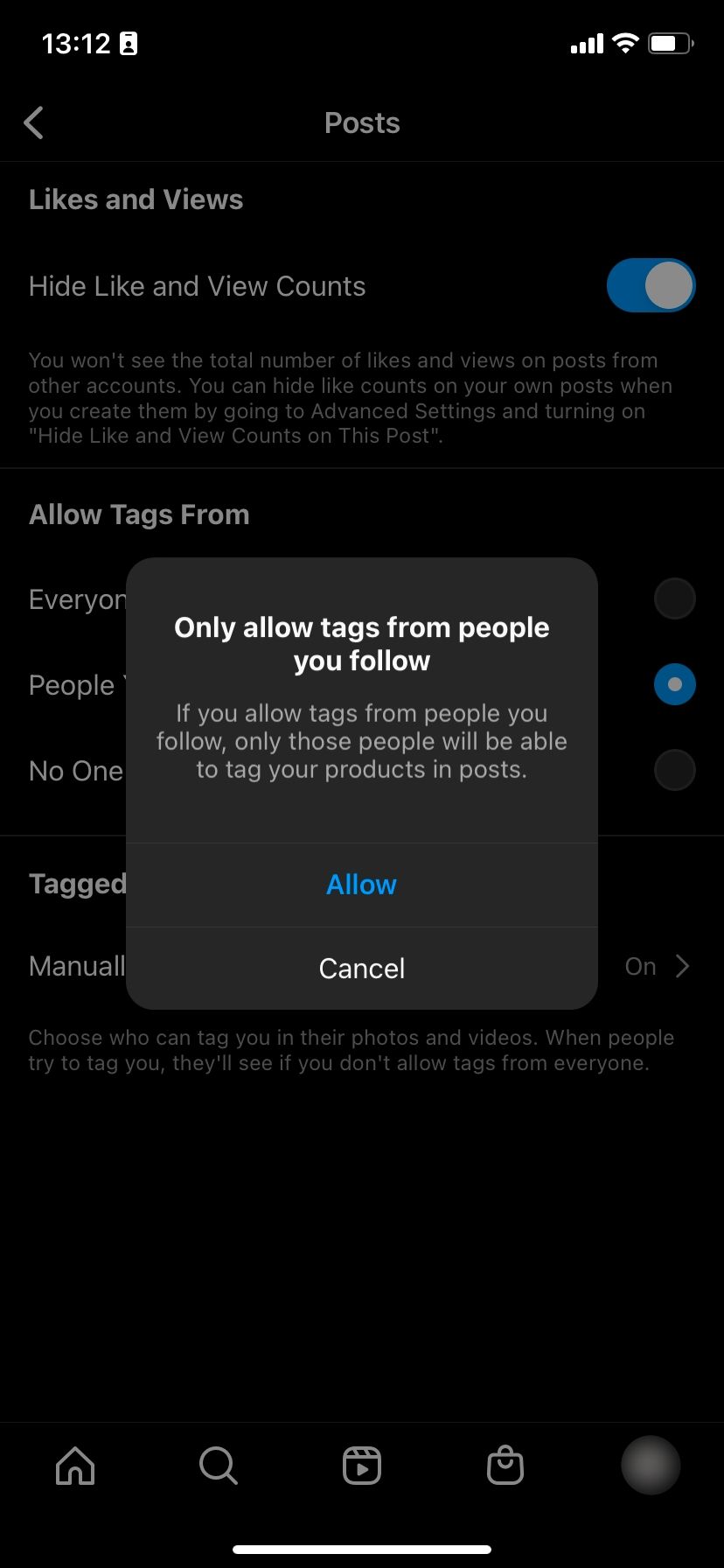Screenshot of an iPhone Interface with Privacy Settings

This image captures a screenshot from what appears to be an iPhone, showcasing its dark theme interface with a black background. At the top of the screen, the time is displayed as 13:12. To the right of the time, the device shows full cell service with four bars, a strong Wi-Fi connection, and approximately 75% battery life.

Immediately below the status indicators, there is a left-pointing arrow icon for navigation, followed by the text "Posts" in gray on the black background. Further down, a setting reads "Likes and Views" with a toggle switch next to it. The switch is activated, indicated by its blue color, showing that the user has chosen to hide their like and view counts.

Dominating the center of the screen is a gray pop-up prompt stating, "Only allow tags from people you follow. If you allow tags from people you follow, only those people will be able to tag your products in posts." Below this message, there are two options: "Allow" in blue text positioned above "Cancel" in white text.

At the bottom of the screen, a row of icons is visible, representing Home, Search, Video, and another unidentified function.